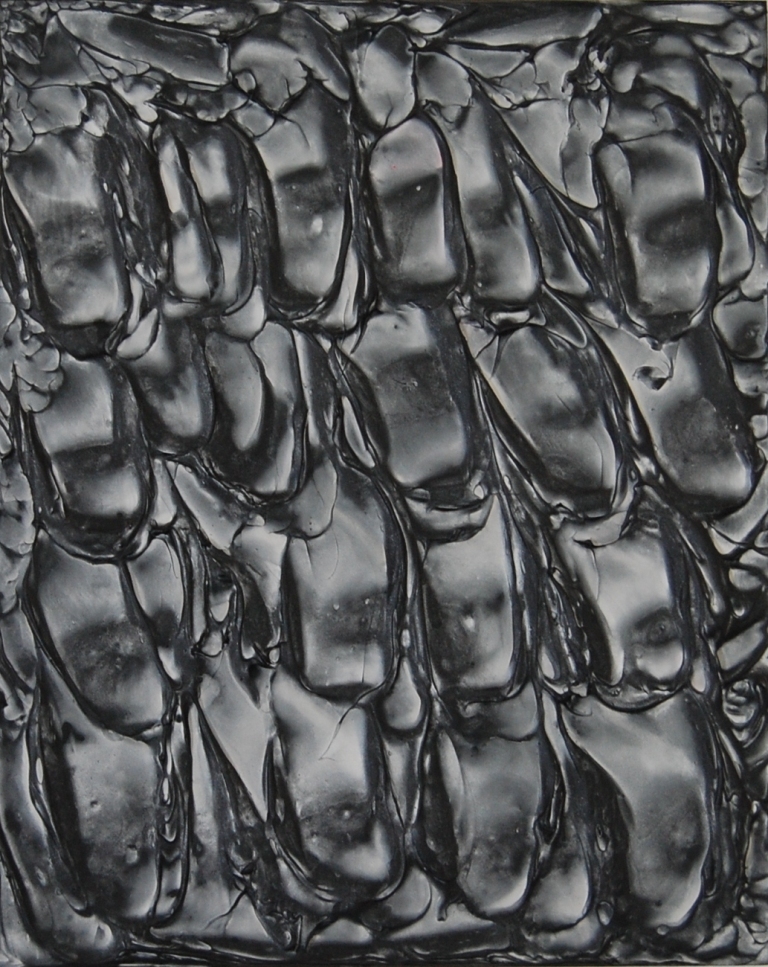The image depicts an abstract scene dominated by a dark, shiny material that can be described as either very dark gray or black. The material is layered and gathered in a three-dimensional manner, creating a bumpy, textured surface. The arrangement is reminiscent of a collection of rectangular and square patches, similar to shingles on a roof. Each patch varies in shape and edge details, with some being wavy, some straight, and others frayed at the top. The material's surface appears to have the appearance of dried oil, with a glossy, leathery finish. The overlapping layers create a complex texture that looks like dragon scales or cooled lava on a canvas, adding a rich, tactile feel to the abstract composition.